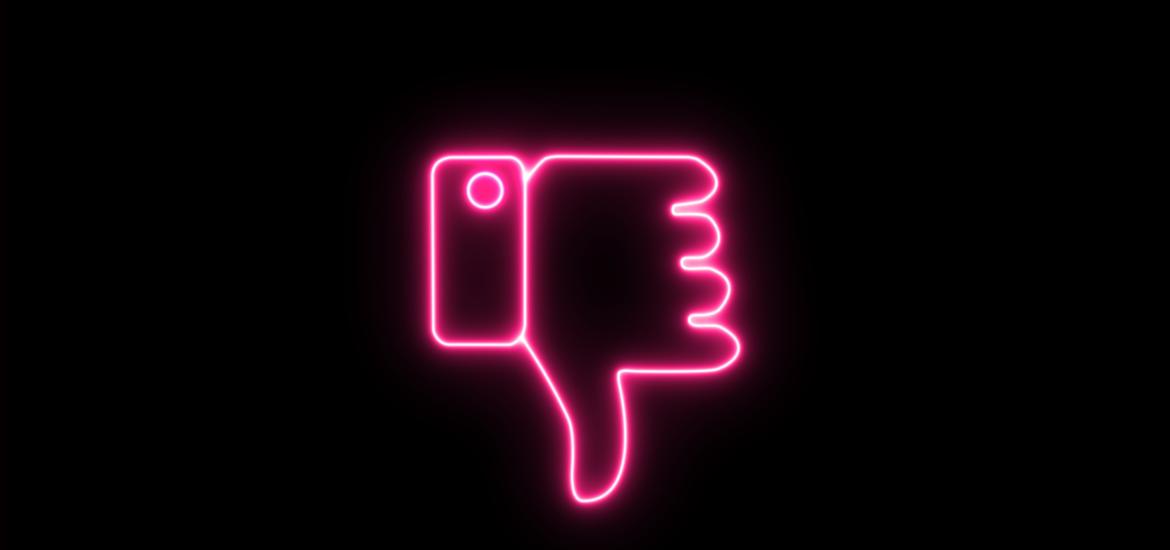In this striking image, a neon light effect portrays the outline of a mechanical-looking left hand against a completely solid black background. The hand, rendered with a consistent and precise white line that glows a vivid pink, has its thumb prominently pointing downward, while the top knuckles of the four curled fingers are visible. The depiction includes a shirt sleeve with a round cuff link where the wrist would be. The neon pink light is sharply highlighted against the dark backdrop, making it the most eye-catching element of the composition. The design is clean and meticulously detailed, giving the impression of a modern, almost digital artwork.